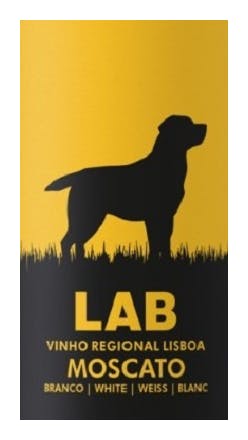The image is a vertically rectangular, two-color print poster featuring a detailed and artistic depiction of a dog in black and gold tones. The top half of the poster is gold, resembling a sky, and features the silhouette of an erect, short-ish tailed labrador dog facing to the right, with flat muzzle and short, floppy ears. The dog is standing in a field of black blades of grass that extends upwards from the bottom half of the poster, which is entirely black. This black area contains text in bold, large yellow letters stating "Lab." Below that in smaller lettering, it reads "Vinho Regional Lisboa," followed by "Moscato," and then the word "white" repeated in different languages separated by vertical lines. The poster appears to be an advertisement for a type of Moscato wine, using the labrador dog as its emblematic figure.